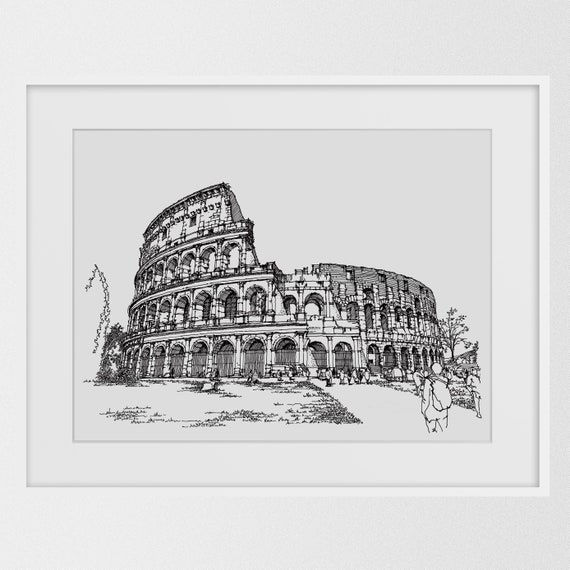This black and white drawing depicts a partially crumbled Roman Colosseum with intricate details. The upper right corner of the structure is notably decayed, showcasing broken arc-like patterns and numerous windows in various states of disrepair. Surrounding the Colosseum are several trees and bushes scattered around, adding to the context of ruin and nature encroaching. At the bottom of the image, a patch of grass and debris can be seen along with a sidewalk leading up to the ancient structure. In the foreground, two people are present: one stands with a backpack, gazing intensely at the Colosseum, while the other is bent over, possibly taking a photo or examining something. The entire scene sits within a white striped border, with a clear, blank sky overhead.